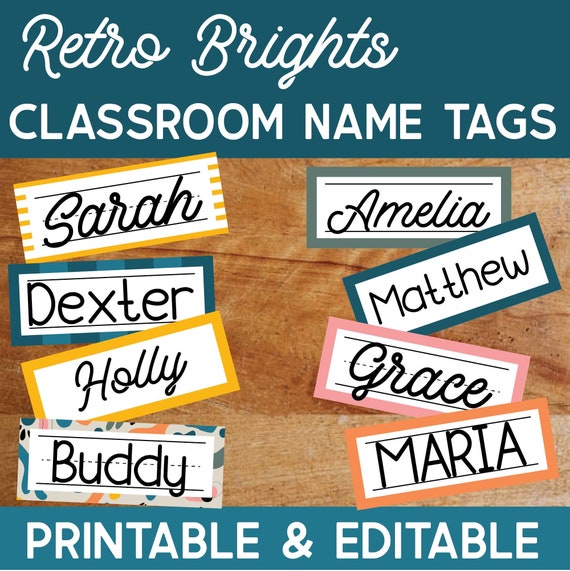This square, illustrated image, resembling a clip art style or an online brochure, features vibrant name tags designed for classrooms. The background showcases a photograph of wooden planks, adding a rustic charm. Across the top of the image, a blue bar with white cursive letters spells out "Retro Brights" while beneath it, in all uppercase letters, "CLASSROOM NAME TAGS" is displayed. At the bottom of the image, another blue bar contains the text "PRINTABLE AND EDITABLE" in white uppercase letters.

The centerpiece of the image exhibits eight distinct name tags, each styled uniquely, arranged in two columns of four. 

- On the left side:
  - The first name tag, sporting an orange border and a traditional handwriting practice line design, reads "Sarah".
  - The second, with a simple white area for writing and a striped blue border, displays the name "Dexter".
  - The third features an orange border with the name "Holly".
  - The fourth, decorated with a colorful, cut-out shapes border inspired by Monet, also uses the dashed handwriting lines and the name "Buddy".

- On the right side:
  - The top name tag, bordered in gray, has "Amelia" written on it.
  - The second tag has a solid blue border with "Matthew".
  - The third tag, with a pink border and handwriting practice lines, reads "Grace".
  - The final name tag features a cantaloupe orange border with the name "Maria".

The names on these tags are a mix of different styles, including cursive, printed, all caps, and regular text, showcasing their editable nature.